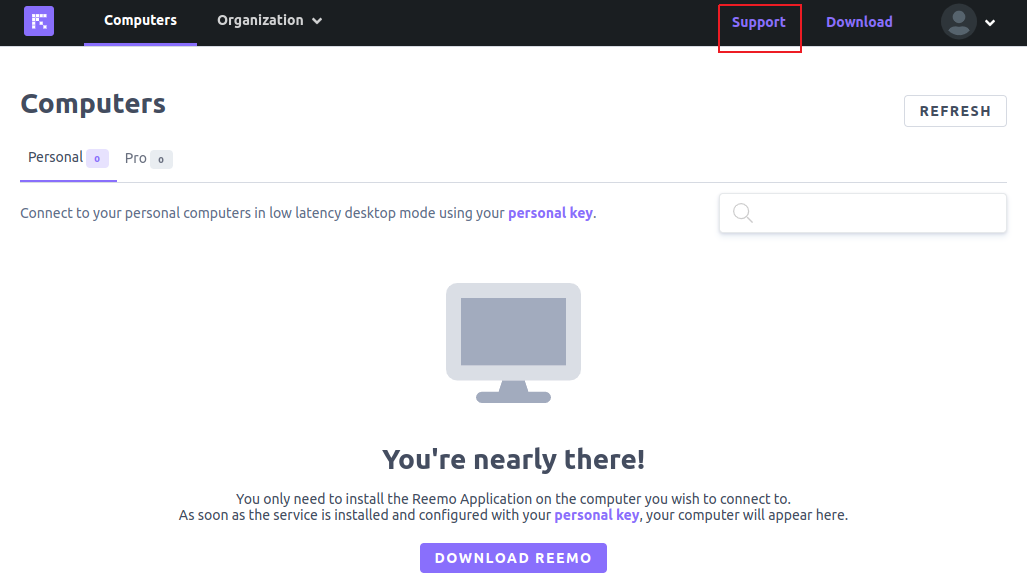This is a detailed screenshot of a computer interface. At the top of the screen, a black horizontal bar spans across, with a purple square in the left corner. Inside this purple box, a white arrow points diagonally up to the left, and the arrow's stem is dashed. Immediately to the right, in white text, the word "computers" is displayed, followed by the word "organization," which features a downward arrow resembling a lowercase 'v.'

On the far right side of this top bar, the words "support" and "download" are written in purple, with "support" being outlined by a red rectangular border. Further to the right, there is a gray profile icon, composed of a gray circle above a gray half-circle, accompanied by a white downward arrow that also resembles a lowercase 'v'.

Just below this top bar, in the upper left corner, the word "computers" appears in large gray letters. Beneath that, the words "personal" and "pro" are displayed, with "personal" on the left and "pro" directly to the right. On the right side of this section, the word "refresh" is enclosed in a light gray rectangle. A gray line, transitioning to purple on the left end, spans horizontally across the screen.

Underneath this line, the text instructs, "connect to your personal computer in low latency desktop mode using your personal key." Centrally aligned below this message is a gray graphic of a computer monitor. Directly below this image, bold black text reads, "you're nearly there." Two lines further down, the text states, "you only need to install the remote application on the computer you wish to connect to." Following this, it mentions, "as soon as the service is installed and configured with your personal key," where "personal key" is highlighted in purple, "your computer will appear here."

Finally, at the bottom of the screen, there is a purple rectangle with the text "download remote" in white font.